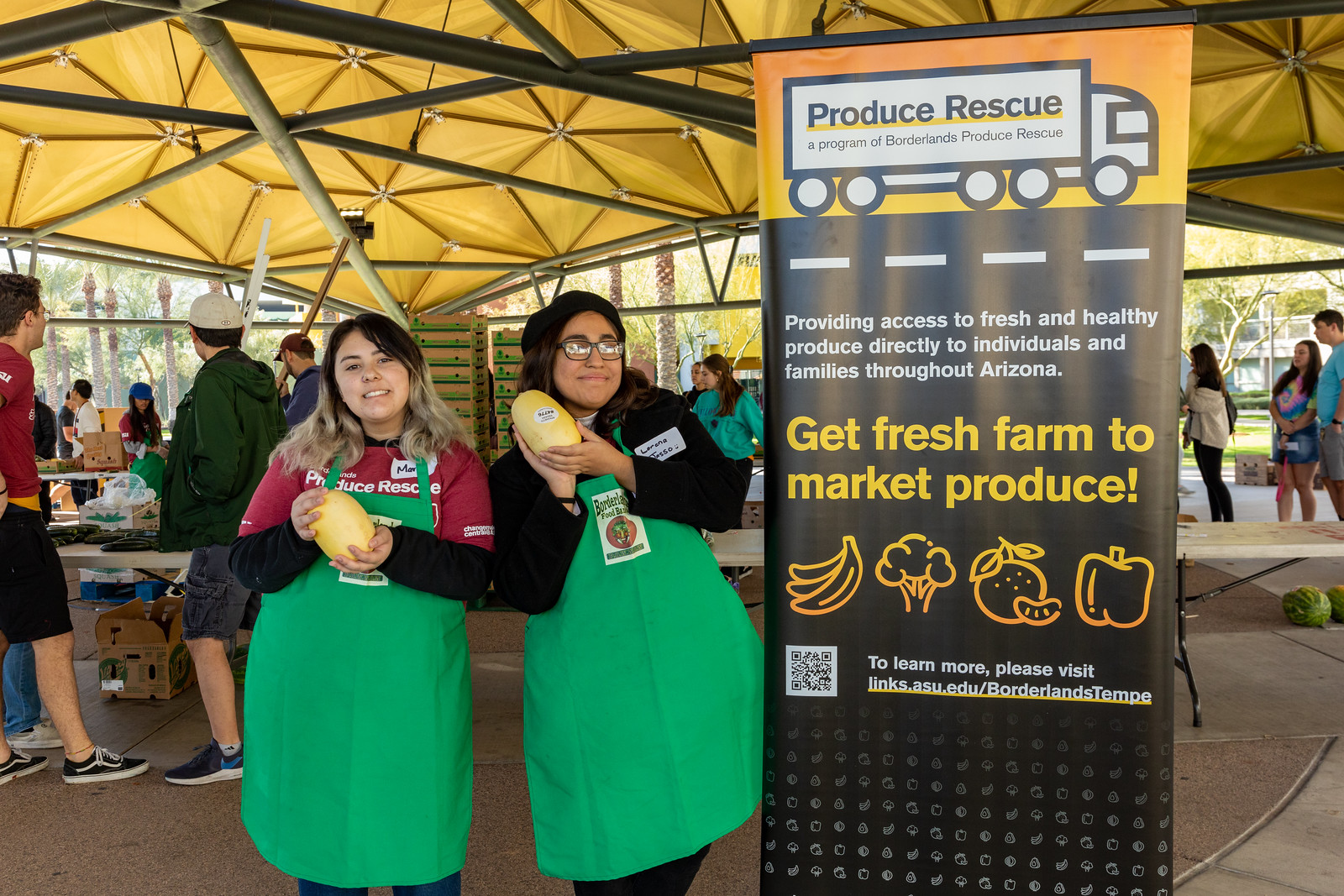In this horizontally aligned rectangular image, two women are featured standing under a yellow tent supported with bamboo-like structures, typical of a farmer's market setup. Both women are wearing green aprons over black long-sleeved shirts. The woman on the left, who has blondish-brown wavy hair cascading over her shoulders, is also wearing a red shirt over her black sleeves and has a partially visible name tag. She holds a large yellow squash in her hands and is smiling. The woman on the right, who wears glasses and a hat, also has long brown hair and holds a similar yellow squash, smiling as well.

Behind them, the bustling market scene includes people dressed in various colors like green, red, blue, and tie-dye shirts, browsing tables with an array of produce. To the right of the image, a tall sign reads "Produce Rescue," part of the Borderlands Produce Rescue program, which provides access to fresh and healthy produce for individuals and families throughout Arizona. The sign itself features white text on a brown background and emphasizes “Get Fresh Farm to Market Produce” in larger yellow text. Below the text are symbols of a banana, broccoli, an orange, and a pepper, as well as a QR code that directs viewers to learn more through a link to asu.edu.